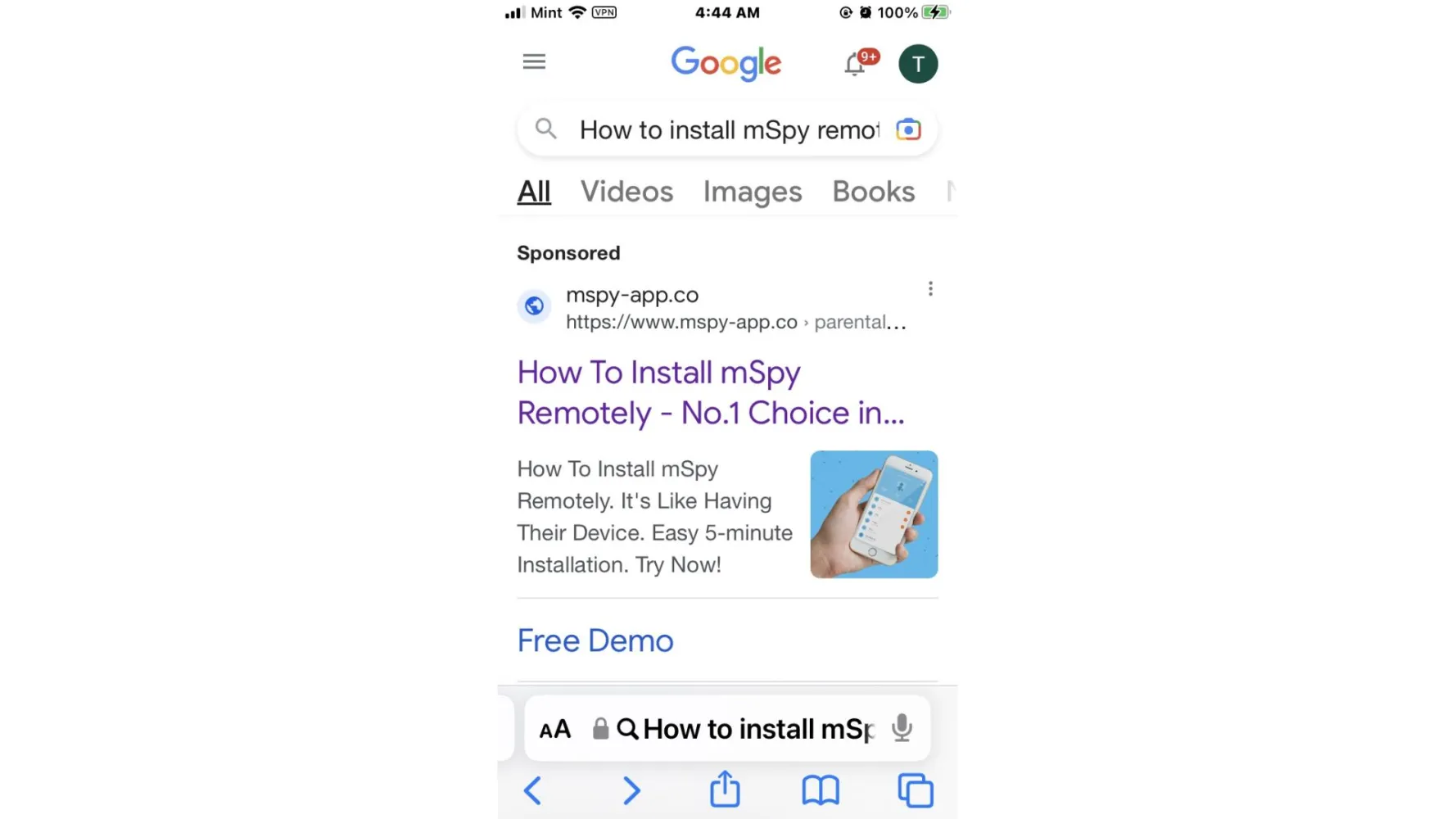The screenshot captures a Google search result page on a smartphone displaying decent reception with three out of four service bars. The phone's status bar shows the carrier as "MIT" alongside indicators for VPN connectivity and a full battery at 100%. The time is 4:44:48 AM, with an active alarm clock icon. 

Below the status bar, the Google search interface is visible. The top-left corner has a triple-line menu icon. Nearby, there's a notifications bell icon, grey with a red oval displaying "9+". Next to it, a green circle with a white 'T' and a white oval featuring a grey magnifying glass are seen, alongside the text "HiTool Store, My M-Spy" in black. 

The primary navigation tabs below this include 'All' (bolded and black), 'Videos', 'Images', and 'Books' (all in dark grey). A thin grey line separates these tabs from the sponsored search results. 

Highlighted prominently is a sponsored link from "mspy-app.co," shown in purple indicating it has been clicked before. It features a blue circle with an Earth symbol followed by the title, "How to Install M-Spy Remotely - #1 Choice". The detailed snippet reads, "How to Install M-Spy Remotely. It's like having their device. Easy five-minute installation, try now." Below this, a blue link offers a "Free Demo".